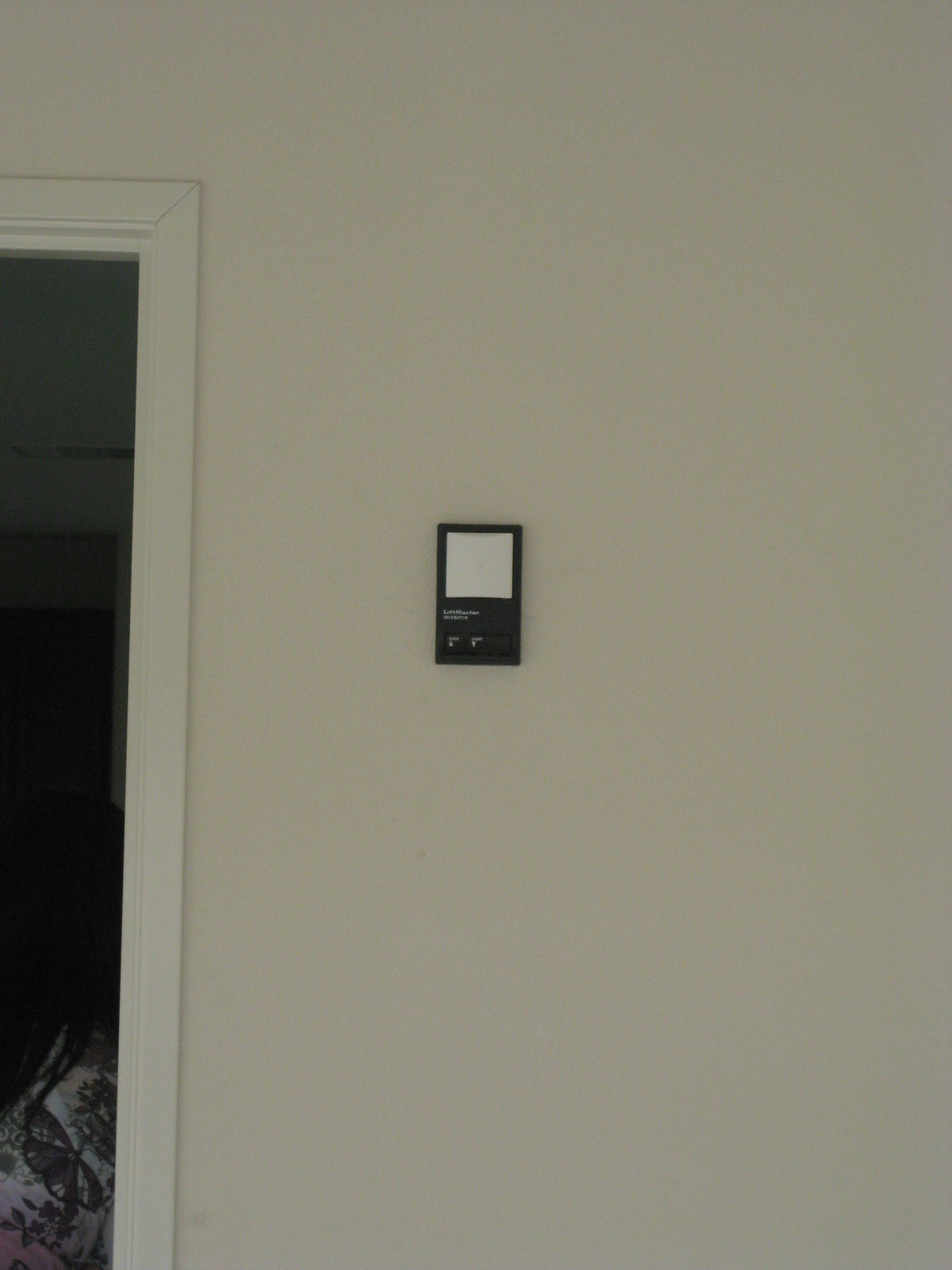The image features a LiftMaster garage door opener mounted on a white or off-white wall. The opener is a rectangular black device with a large white square button at the top, followed by two smaller buttons beneath it. The brand name "LiftMaster" is prominently displayed between the large button and the smaller ones, with an additional word underneath that is not legible. The wall to which the opener is attached is slightly darker than the off-white door trim visible on the left side of the image. The partially visible door leads into a dimly lit room where the edge of a piece of furniture, possibly a bed with a white comforter adorned with butterfly or floral designs, can be seen. The two smaller buttons on the opener appear to have symbols resembling light bulbs and are labeled "Lights," suggesting they control the lighting. Besides the garage door opener, the image does not contain any other significant elements.